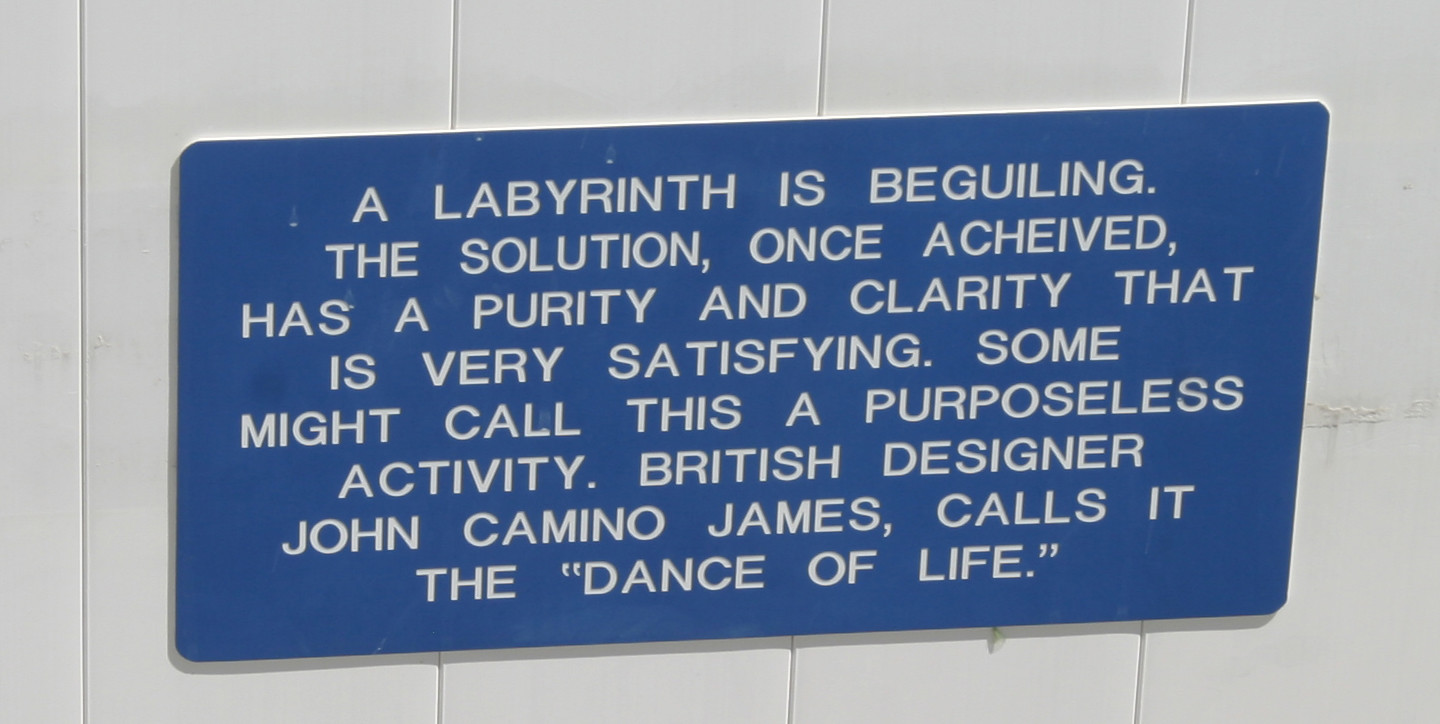The image depicts a blue rectangular sign mounted on a wall composed of white tiles. The sign features white, all-capitalized text. It displays a quote that reads, "A LABYRINTH IS BEGUILING. THE SOLUTION, ONCE ACHIEVED, HAS A PURITY AND CLARITY THAT IS VERY SATISFYING. SOME MIGHT CALL THIS A PURPOSELESS ACTIVITY. BRITISH DESIGNER JOHN CAMINO JAMES CALLS IT THE 'DANCE OF LIFE.'" The blue rectangular sign has a medium blue background with slightly curved corners, and its width is greater than its height.